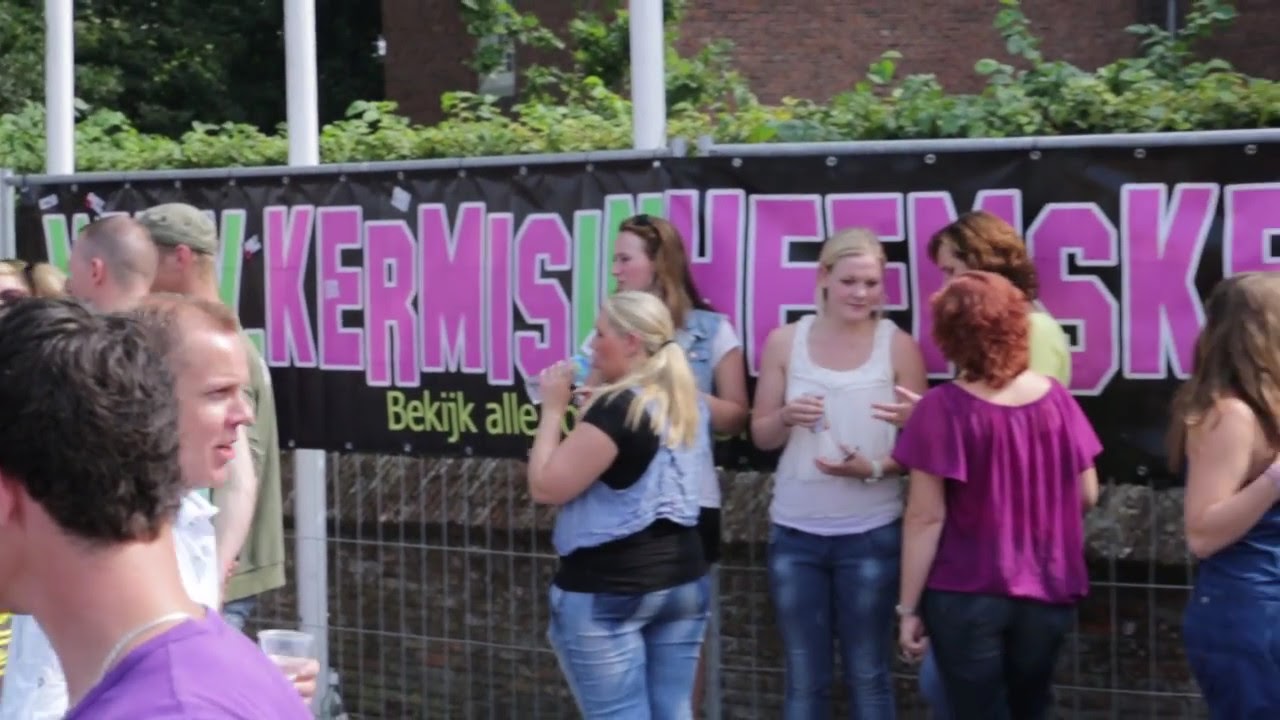In this full-color outdoor photograph taken on a sunny day, a group of mostly young Caucasian women and a few men are standing around at what appears to be an event, possibly a school-related gathering or a small festival. The image is horizontally rectangular, capturing a bustling yet casual scene. 

The people are dressed in light blue, white, magenta, and purple outfits, predominantly in short-sleeved shirts and blue jeans, suggesting the weather is pleasant but not overly warm. The women are clustered in the center and right side of the image; many have water bottles in their hands. The men, meanwhile, are mostly situated on the left. One man wears a purple shirt, and another has a green cap.

A black banner with colorful text, predominantly in pink and green letters bordered by white, stretches across the fence behind the group. The text is in a non-English language, possibly Swedish or a similar language. The visible letters include "K-E-R-M-I-S-H-E-E-N-S-K" and "B-E-K-N-K." Behind the fence, lush green bushes and a brick building add depth to the background.

Overall, the cheerful atmosphere, informal clothing, and speculative educational context set the scene for a lively event among friends or acquaintances.